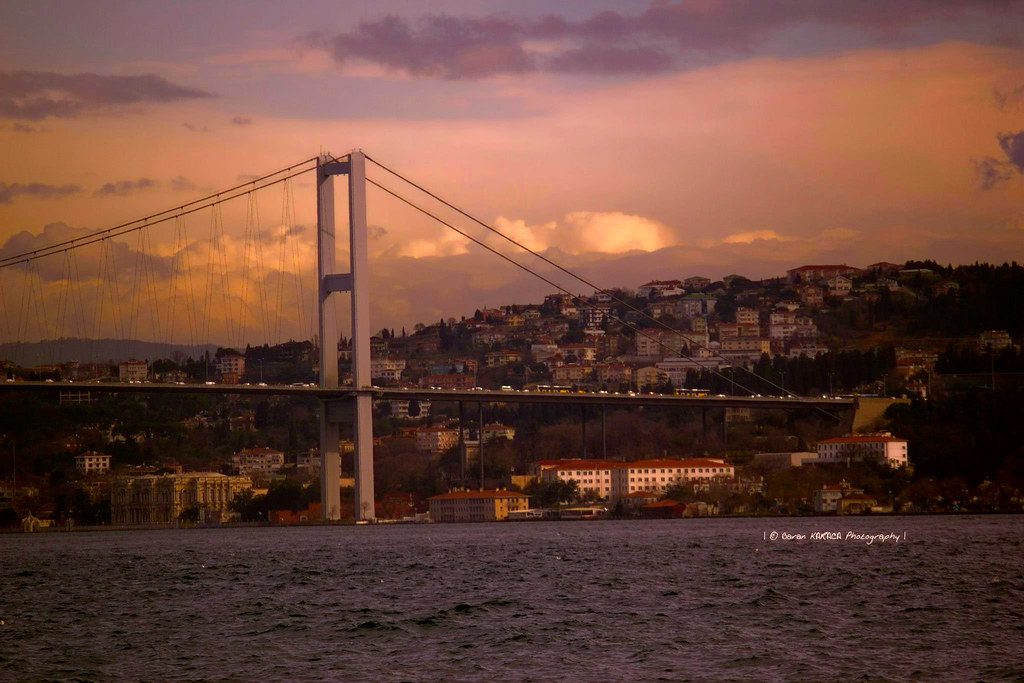In this rectangular photograph, a graceful white suspension bridge stretches across a choppy, blue body of water. The forefront of the image features numerous car headlights, illuminating the bridge and highlighting the bustling activity. Large black wires support the bridge, towering into the vibrant sky, which is painted with warm orange hues indicative of a sunset, dotted with occasional clouds.

In the backdrop, a scenic hill is densely packed with small houses, their roofs a mix of red and white, evoking a sense of an upscale neighborhood. This picturesque view hints at a familiar, possibly iconic, cityscape resembling areas like Istanbul or San Francisco. Trees and brush pepper the landscape, adding to the depth and realism of this outdoor scene.

Impulsing over the water in the lower part of the photograph is a white text watermark that reads "copyright Karen Kakaka photography." Despite the rich detail, no boats traverse the water, focusing the viewer’s attention on the bridge and the vibrant life it carries. The warm sunset colors and the detailed, photorealistic depiction amplify the serene yet dynamic quality of this captivating scene.